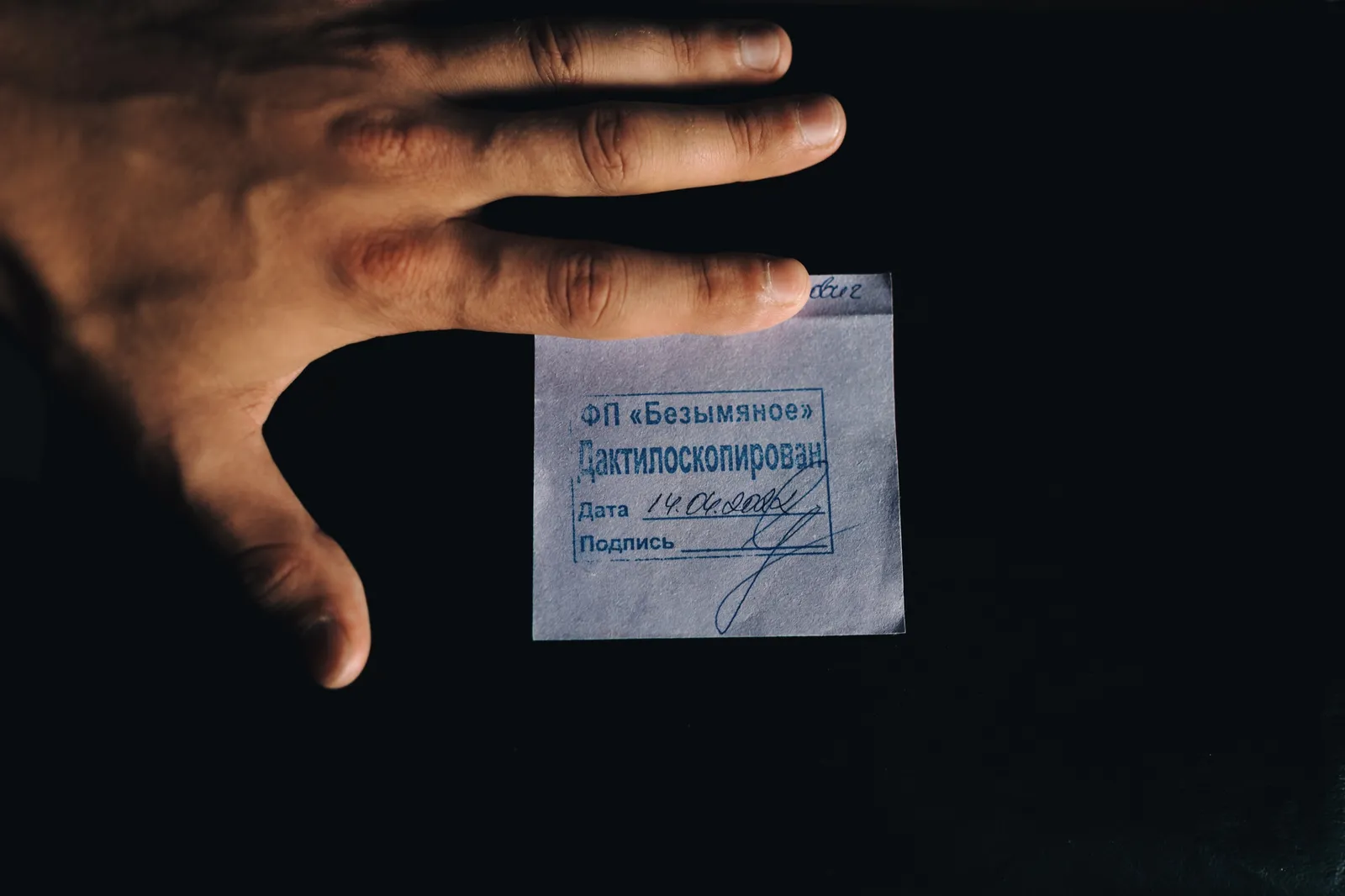In this evocative photograph, a well-manicured left hand is firmly planted against an intensely dark, pure black background. The hand has a natural appearance with visible veins and various markings, and the pinky finger is not shown. The thumb and three other fingers are spread out, with the pointer finger pressing down on a small, white square piece of paper. This piece of paper, likely a post-it note, features blue text and characters that appear to be in Russian, including the letters G-A-K-T-N-O-C-K-O-H-P-O-B-A-H, indicating it could be for legal or mailing purposes. There is also an inked stamp on the paper and a somewhat illegible handwritten signature beside the letters A-T-A. The hand’s firm placement suggests it is securing the note in place on the dark surface.